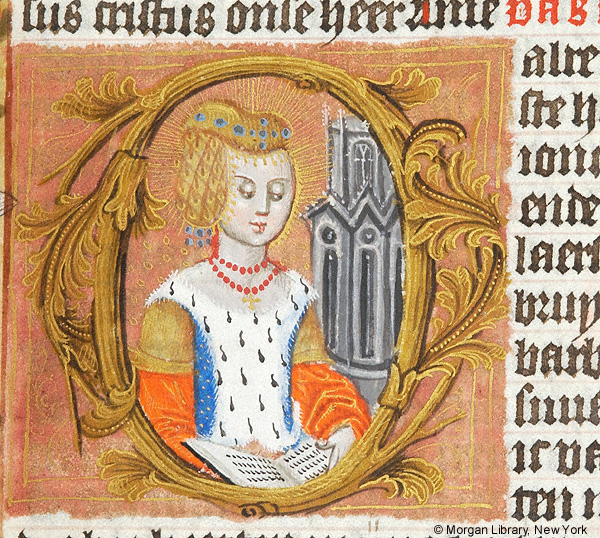The image depicts an old, detailed illustration of a young woman, designed like a medieval or Renaissance character. She appears to be reading a book with indistinct black lines representing text. The woman, possibly a noble or scholar, is adorned with a red beaded necklace featuring a yellow cross, black marks on her white bodice resembling musical notes, and additional blue fabric with gold accents. Her puffy sleeves transition from white with orange to gold-tinged fabric near her shoulders. She has blond hair, styled and contained in a golden net. Around the entire scene is an ornate frame decorated with floral and plant designs, possibly including elements like corn or fleurs-de-lis, in gold. This frame is bordered by text resembling Hebrew or some other ancient script. In the background, there is a cathedral tower or castle depicted in gray. The scene is set against a pinkish-beige background with the image contained within a dark orange square. Overlay text at the bottom reads "Morgan Library New York, New York."